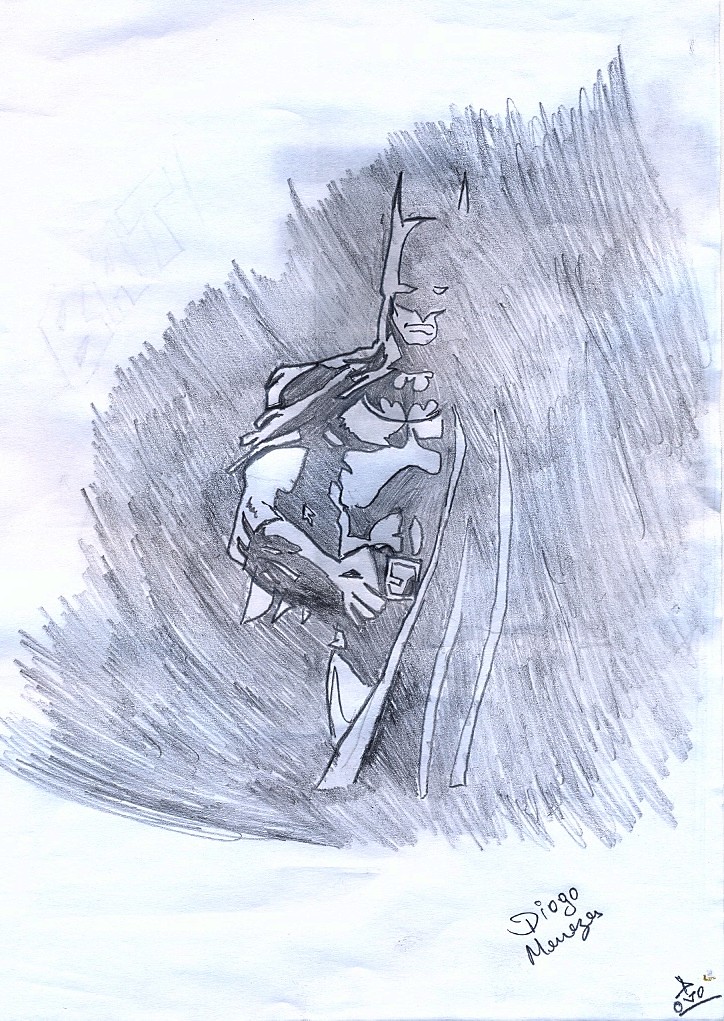This is a highly detailed, vertical, and rectangular color photograph of an intricate pencil sketch of Batman, attributed to Diogo Menezes. The character is rendered predominantly in blue, gray, and black hues. The sketch captures Batman from the top upper right down to about three-quarters of the frame, primarily focusing on his left side. Batman is depicted with his iconic pointy-eared mask, which covers his forehead and eyes but leaves his mouth visible. His right shoulder is obscured, and his right arm is shown almost touching his belt buckle.

The background features a diffused, sky-like ambiance with light shades of white, blue, and gray. Faint block letters spelling “B-A-T” are visible diagonally on the upper left side. Batman’s suit includes notable details such as his black bat emblem on the chest, gray gloves with two spikes on the forearms, and a flowing gray cape.

At the bottom of the image, the artist’s signature is present, reading "Diogo Menezes," with some letters appearing scribbly. Additionally, the lower right corner contains an enigmatic symbol that looks like an '8' next to "05 0" with a line drawn beneath it. The detailed pencil strokes and shading emphasize the depth and intensity of Batman’s figure, creating a vivid and striking representation of the superhero.